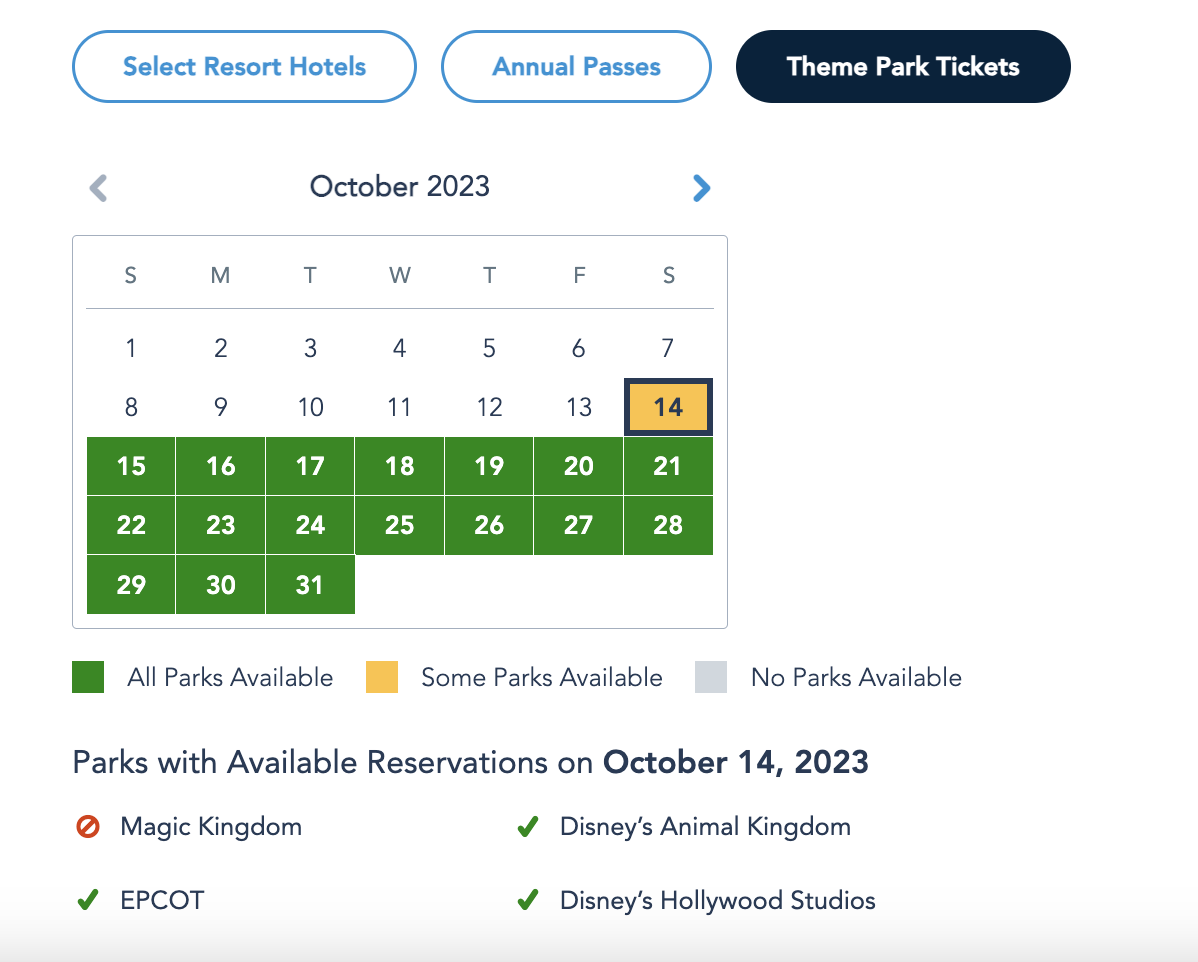The image shows a detailed calendar for October 2023, specifically depicting the availability of select resort hotels, annual passes, and theme park tickets. The dates from the 1st to 13th are displayed in white with black numerals, indicating a baseline status. On October 14th, the date is highlighted in orange with a black square, drawing attention to it. Dates from the 15th to the 31st are marked in green with white numbers, signifying full availability at all parks.

Key:
- Green: All parks available
- Yellow: Some parks available
- Gray: No parks available

For October 14, 2023, the reservation status for each park is as follows:
- Magic Kingdom: No reservations available
- Epcot: Reservations available
- Disney's Animal Kingdom: Reservations available
- Disney's Hollywood Studios: Reservations available

This visual guide helps potential visitors understand park access and plan their trips accordingly.